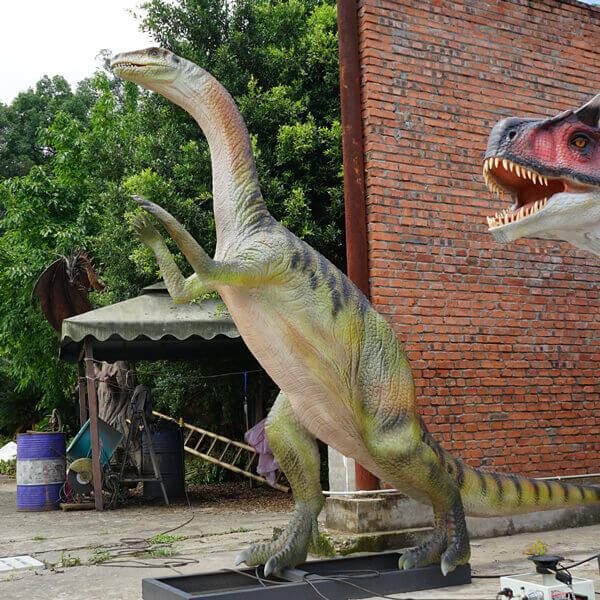The image features a large statue depicting a dinosaur, standing upright on its hind legs on a rectangular black metal platform. The dinosaur is predominantly green with black stripes along its body and tail, and bears a tan underbelly. Its small front arms are bent at the elbow and held up. The creature has a long, upright neck with a brownish side and tan underside, leading to a small head reminiscent of a snake. The dinosaur also has three prominent toes with sharp nails on its dark green feet. 

To the right of this main dinosaur, the head of another dinosaur is visible, characterized by its red and black coloring, white underside of the chin, and open mouth showing sharp, pointy teeth. In the background, there is a tall brick wall with a thin profile, beyond which a canopy or gazebo with brown wooden legs and a light gray top can be seen. Underneath the canopy, various items, including a fallen ladder, are scattered. There is also a distinctive blue and white striped barrel next to a green bucket. Surrounding the scene are numerous trees, adding lush greenery to the background.